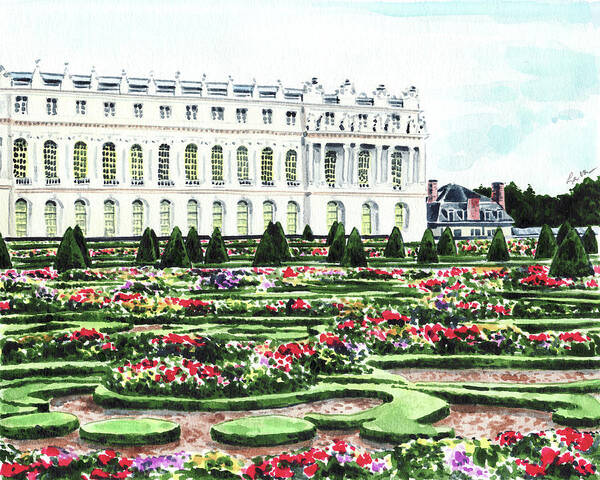The image portrays a hyper-realistic watercolor painting of a grand European estate. Dominating the scene is a large, white, castle-like building, stretching horizontally with an array of windows repeating uniformly, featuring tiny square windows on the top floor and multiple arched windows on the lower floors. To the right, a smaller building with a rounded roof and three red chimneys stands in contrast yet complements the grand structure. 

In the foreground, an impeccably maintained garden displays a vibrant tapestry of red, purple, and yellow flowers. The garden is adorned with low, hedge-like shrubs designed in intricate patterns and interspersed with orderly planted trees and bushes. The grassy areas are meticulously cut into circular and weaving designs, adding depth and interest to the floral display. Above, a light blue sky frames the idyllic daytime scene, adding a serene backdrop to the richly colored and highly detailed landscape.